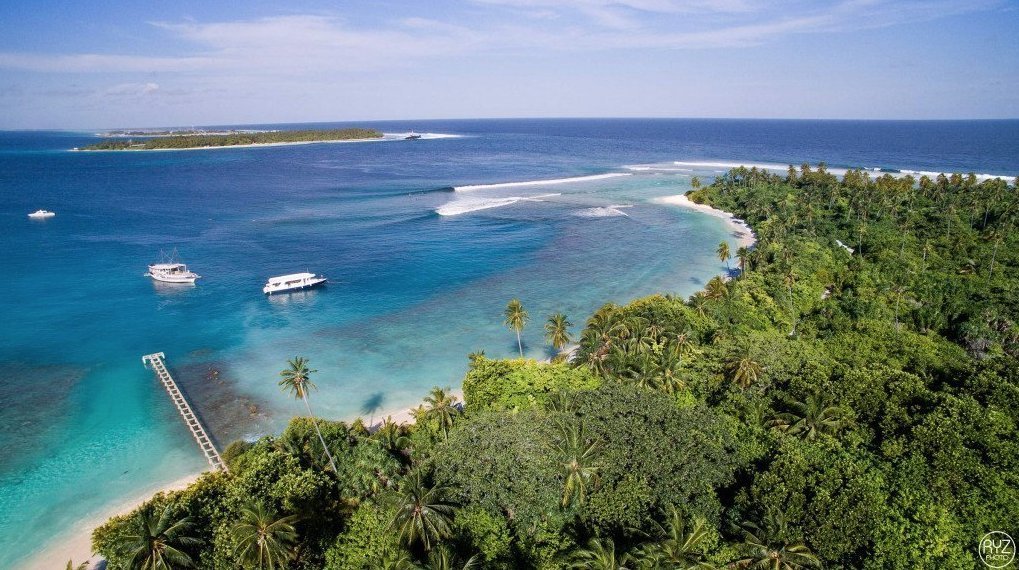In this stunning horizontal seascape, a panoramic view of a tropical paradise unfolds before the viewer. The photograph captures a broad expanse of a teal-colored ocean under a partially clouded, azure sky. To the left, an island blanketed with vibrant green palm trees curves gently into the crystalline bay. In the foreground, a golden, light-sand beach stretches out, adorned by a jetty extending into the tranquil waters from the bottom left corner.

A few boats are peacefully anchored in the bay, their silhouettes adding a sense of scale and tranquility to the scene. The photo seems to be taken from an elevated vantage point, possibly atop a hill or a tall structure on the island, offering a sweeping view of the landscape below.

Dominating the center of the image, waves can be seen gracefully crashing against the shoreline on the right side of the bay, near a breakwater that arcs gracefully into the sea before curving back towards the land. Beyond this serene island bay, the vast, inviting ocean stretches out towards the horizon. This radiant tropical haven, with its lush palm trees, pristine white beach, and clear sunny weather, epitomizes an idyllic getaway.